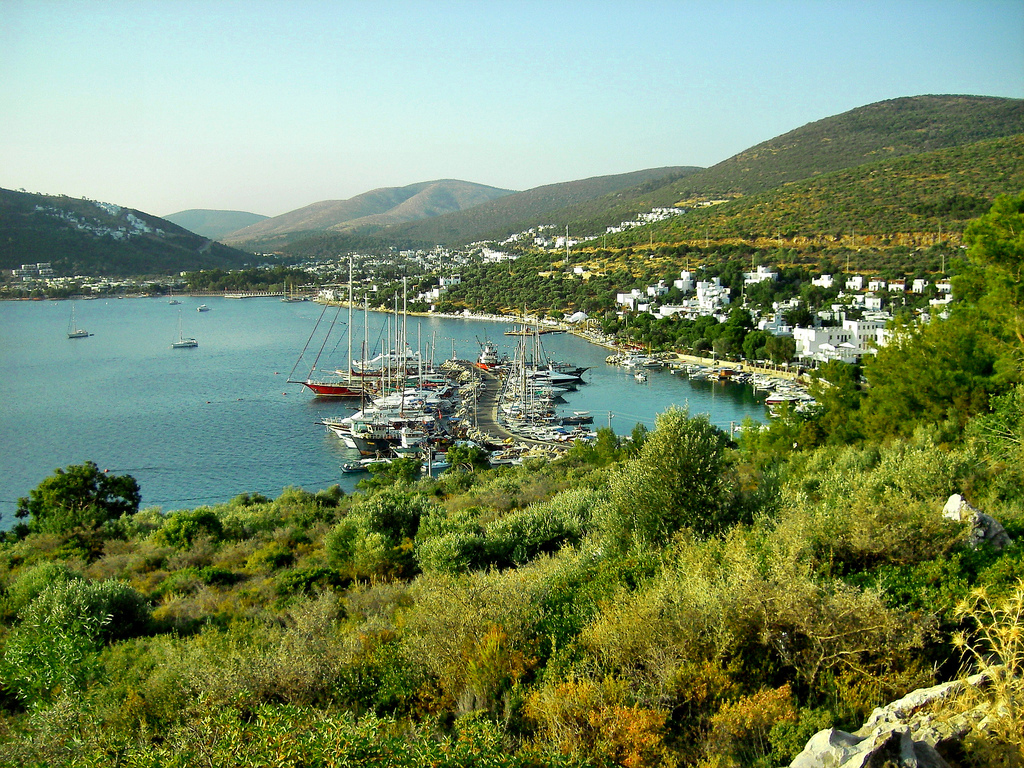This detailed and vibrant image captures a serene Mediterranean marina scene, with mountains and greenery gracing the background. The marina, centrally located in the frame, is a haven for numerous sailboats docked along a long pier, with some boats already out on the calm waters to the left. White houses, consistently painted and architecturally uniform, are scattered across the right side of the image, climbing up gently sloping hills and blending into the lush, tropical greenery that surrounds them. The scene is bathed in warm, sunny light under a clear blue sky, creating a tranquil and inviting atmosphere. To the foreground and right of the image, greenery extends to the water’s edge, enhancing the natural beauty of the landscape. The overall portrayal suggests a peaceful, warm climate, perfect for leisurely sailing and enjoying the picturesque setting.